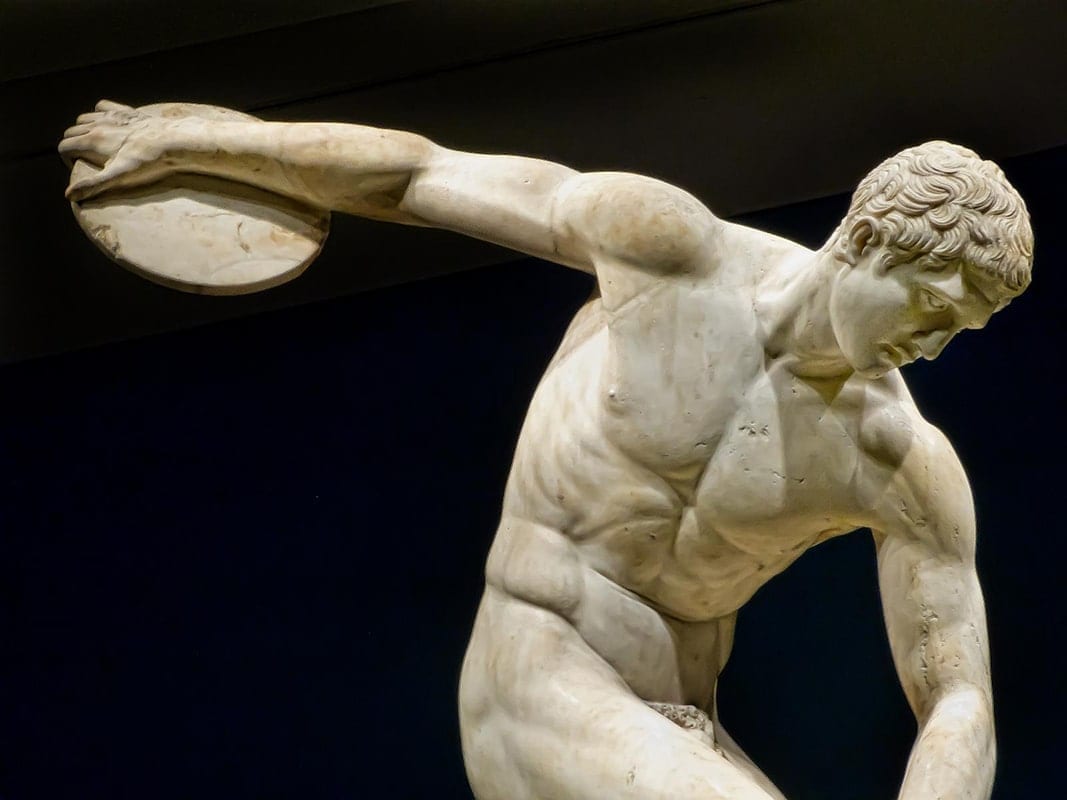The image depicts a highly detailed, realistic marble sculpture of a discus thrower, reminiscent of classical Greek or Roman art, similar to the works from Michelangelo's era. Crafted from white marble, the muscular figure is rendered with exceptional anatomical precision, showcasing a well-defined chest, ripped abs, and pectorals. The athlete stands naked, his curly hair sculpted in dark marble, adding contrast to his form. The discus is held in his right hand, which extends behind his back, creating a dynamic twist in his upper torso that highlights his musculature. His body leans forward, knees bent, capturing the moment just before he releases the discus. His left arm is positioned down by his side. The entire scene is set against a stark black background, emphasizing the sculpture's intricate details and classical beauty.